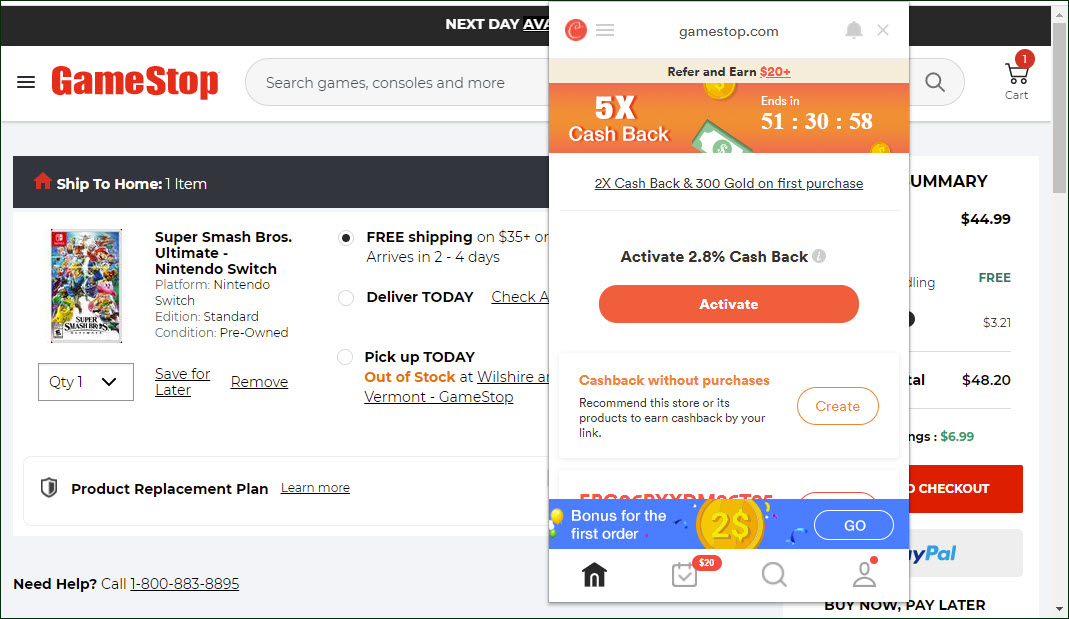The image shows a GameStop checkout page for Super Smash Bros. Ultimate on the Nintendo Switch, with a quantity of one and free shipping. The total cost is $48.20. A prominent red "Go To Checkout" button is located at the bottom of the screen. Slightly right of the center, there is a pop-up offering a cashback credit card deal with 5X cashback and 2.8% cashback, which ends in 51 hours. The remaining elements suggest a white background with the GameStop logo in red, accented by black horizontal bars. There is also an option for "Deliver Today" with an unspecified price and a "Pick Up Today" option that indicates the item is out of stock.